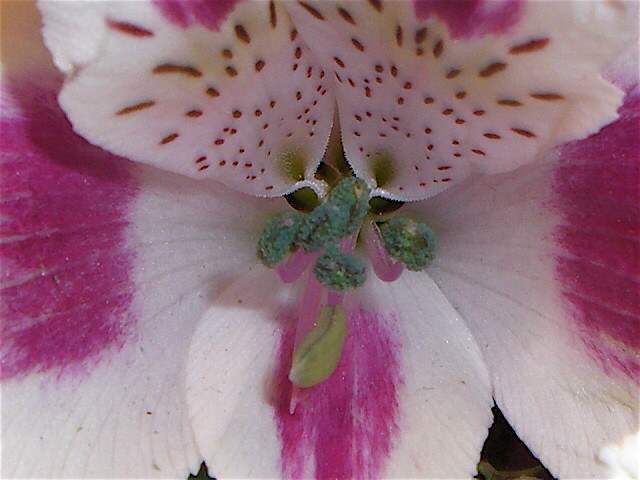This is a perfectly square, close-up photograph of a flower, dominated by its intricate petals and minimal background. The flower has five distinct petals: two at the top, one at the bottom, and two on the sides. The petals are primarily white on the outer edges, transitioning to a dark pink or fuchsia shade toward the center. The two top petals stand out with a scattering of tiny black seeds and a tan background half way down, while the side and bottom petals appear larger, showcasing broader areas of the fuchsia hue. Embedded in the white and pink gradients of the petals are varying pink dots, which coalesce into lines as they reach the petal edges. The heart of the image reveals green stems and small leaf-like structures protruding from the flower's center. Dotted around the flower's core, resembling pink strings or filaments, add delicate intricacy to this vibrant and detailed botanical portrait.